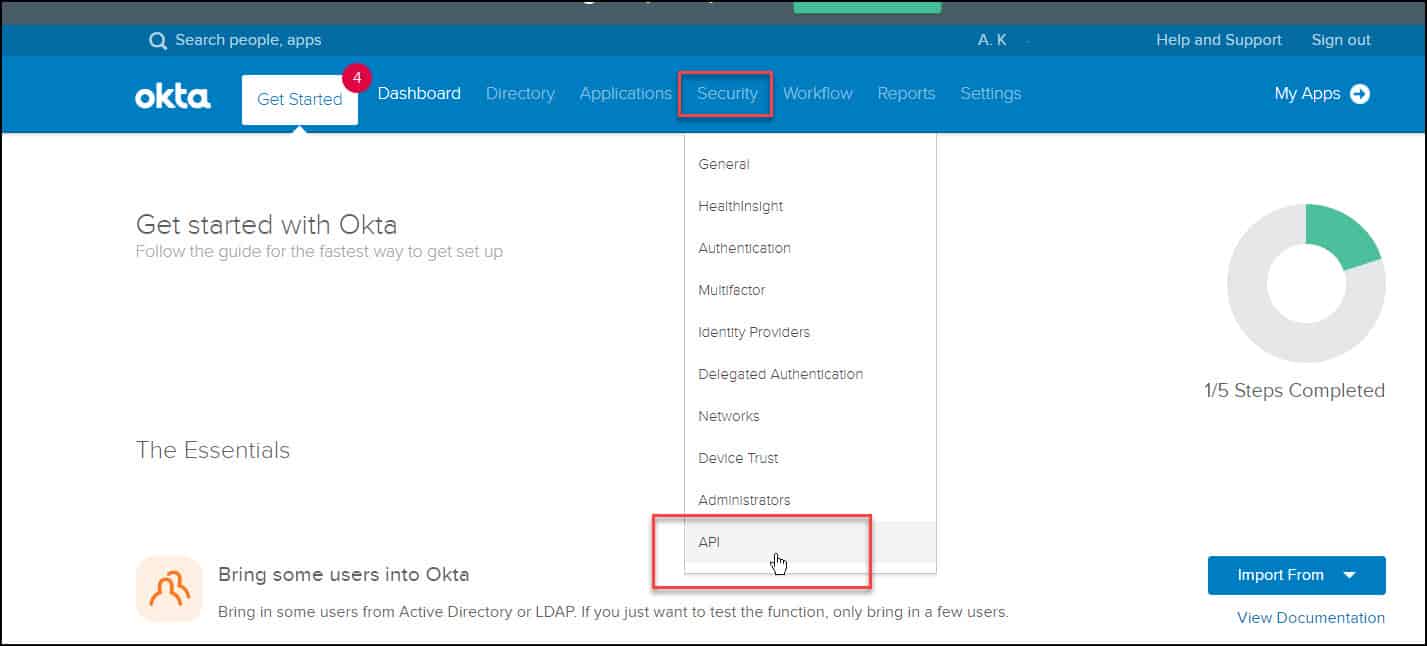The image showcases a user interface of a web application or desktop software from a company called Okta. At the top of the screen, there's a blue navigation bar. On the left of this bar is a search field labeled "Search people apps," while on the right, it features links for "Help and Support" and "Sign Out."

Below this navigation bar, the Okta logo is positioned on the left in white text. Adjacent to the logo are horizontally aligned menu options: "Get Started" (indicated with a white outline and a notification icon showing '4' notifications), "Dashboard," "Directory," "Applications," "Security," "Workflow," "Reports," "Settings," and at the far right, "My Apps." The "Get Started" section appears to be open.

The main window beneath the menu bar has a white background. To the left, the text reads "Get Started with Okta," followed by a smaller text saying "Follow the guide for the fastest way to get set up." Further down, another section titled "The Essentials" is visible. Below this, there's an icon depicting two people and a prompt that reads "Bring some users into Okta." It elaborates, "Bring in some users from Active Directory or LDAP. If you just want to test the function, only bring in a few users."

Towards the center of the screen, a drop-down menu from the "Security" option is open, highlighted with a red outline. This drop-down menu lists several items: "General," "Health Insight," "Authentication," "Multi-factor," "Identity Providers," "Delegated Authentication," "Networks," "Device Trust," "Administrators," and "API," with the latter also marked with a red outline.

On the far right of the main window, there's a progress circle indicating that one-fifth of the steps are completed, with one segment of the circle highlighted in green. At the bottom of the screen, a blue button labeled "Import from" is visible, with an option titled "View Documentation" beneath it.